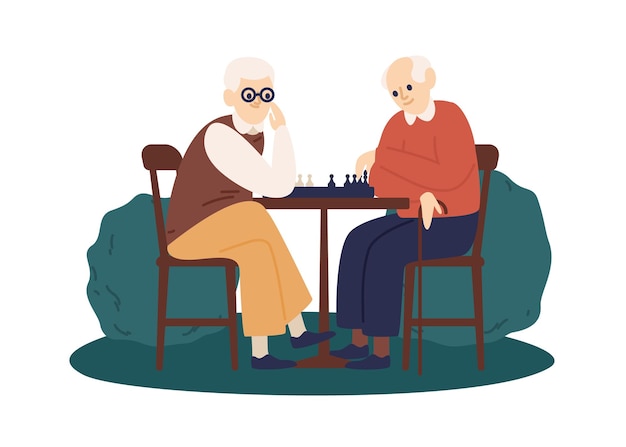This image portrays a simple, cartoon-style scene of two elderly individuals engaged in a game of chess outdoors. The characters, both with white hair, are seated at a wooden table and on wooden chairs, all set on a circular patch of green grass with two abstract, teal-colored bushes in the background. The balding man on the right, dressed in a red shirt with blue pants, brown shoes, and holding a wooden cane, is focused on moving his black chess pieces. The person opposite him, who appears to be a woman, is wearing a brown vest over white sleeves, tan loose slacks or a skirt, and black glasses. Her white hair fully covers her head. Both seem absorbed in the game, conveying a peaceful, thoughtful atmosphere typical of a pleasant day spent in quiet recreation. The background of the image is plain white, devoid of any further details, emphasizing the simplicity and calmness of the moment captured.